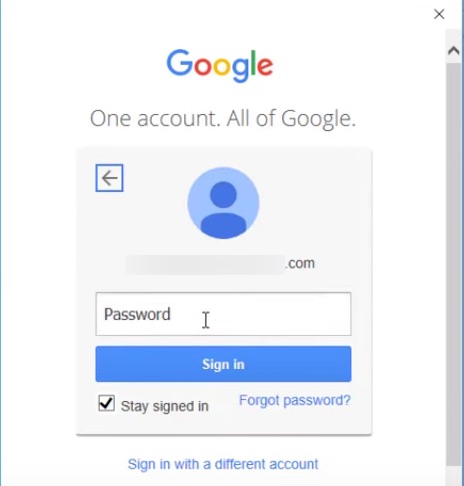The image depicts a Google sign-in pop-up window set against a white background. The pop-up is bordered by thin gray lines on both the left and right sides. On the right side, there is a scroll bar, and in the top right corner, there is a recognizable 'X' icon for closing the pop-up.

At the center of the pop-up is the iconic Google logo, featuring a capital 'G' in blue, a red 'o', a yellow 'o', a lowercase 'g' in blue, a green 'l', and a lowercase 'e' in red. Below the logo is the text "One account. All of Google."

Directly beneath this text is a gray box. In the top left corner of the box, there is a small square with a blue border enclosing a black arrow pointing to the left. Next to this is a blue circle containing the silhouette of a person. Below this circle is an area that has been intentionally blurred, showing partial text that includes ".com".

Further down, there is a text box labeled "Password" where users are to enter their password. Below this text box is a prominent blue button labeled "Sign in."

At the bottom of the pop-up, on the left side, there is the option "Stay signed in" with a checkbox next to it. To the right, there is a blue hyperlink reading "Forgot password?".